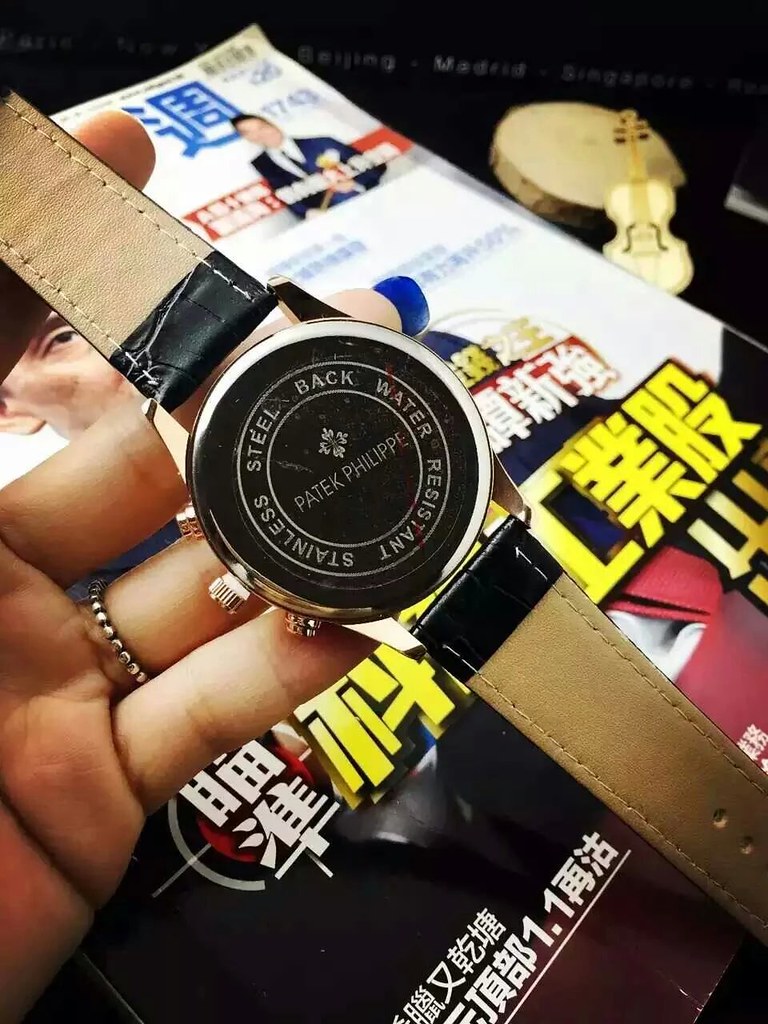In the image, a hand is holding a luxury Patek Philippe watch with its stainless steel backing removed, revealing the intricate internal mechanism. The watch back highlights its water-resistant feature. The watch features a black leather strap with tan stitching, although the leather near the top connection appears wrinkled and slightly damaged, raising questions about its authenticity. The background is a cluttered scene of scattered papers or magazines from an Asian country, adding a sense of everyday life and cultural context to the photograph.